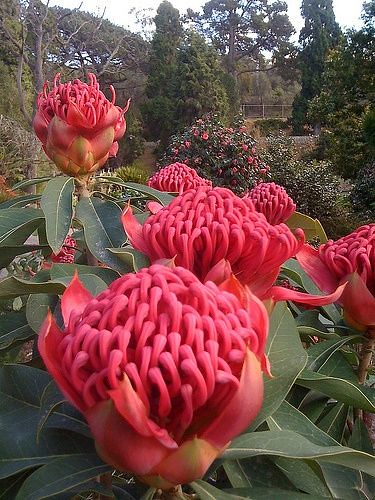In this vibrant outdoor garden scene, the foreground features six large, red flowers with thick petals, each opening up to reveal a multitude of red pistils curling inward, resembling red fingers pointing towards the center. These blooming flowers are surrounded by lush, green leaves that are attached to the same stems or vines from which they grow. Among the varied greenery, other bush-like plants can be seen bearing similar reddish flowers in the middle distance, enhancing the rich tapestry of colors.

The background showcases an array of different trees, including distinctive evergreens with needle-like leaves and a large, bare-branched dead tree standing out for its barren appearance. Amidst this verdant setting, a picturesque arch bridge with a railing traverses the scene more towards the right-hand side, adding architectural interest. The sky above is a light bluish white, suggesting a sunny spring or summer day. The garden boasts a diverse assortment of plant life, creating a striking contrast between the uniform trees within the garden and the more irregular, less uniform trees beyond the garden's fence.